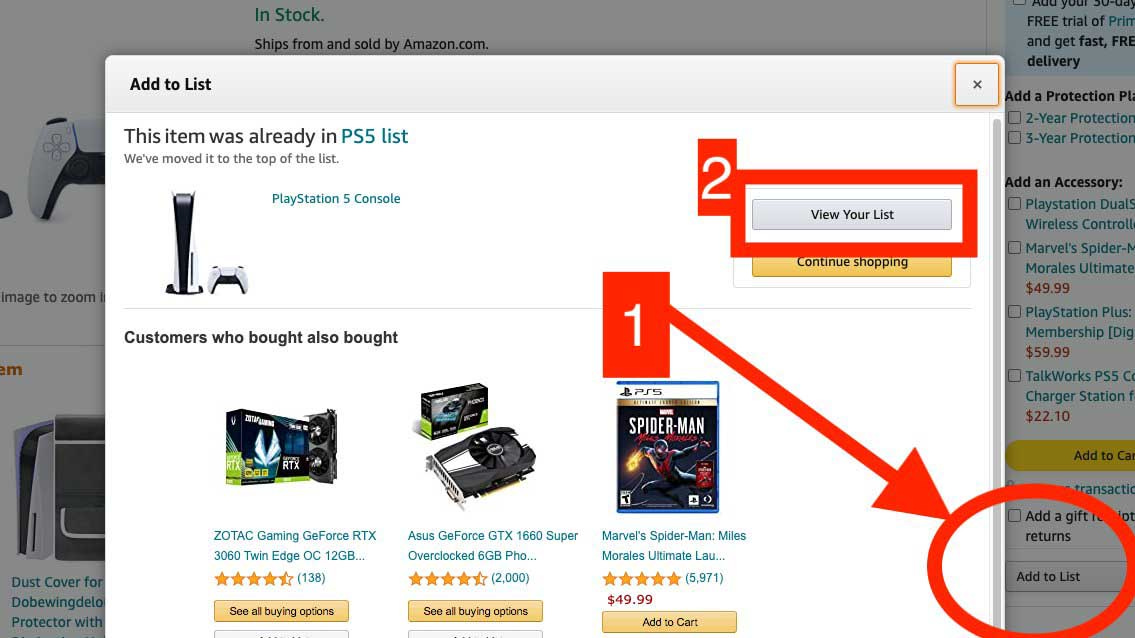A screenshot from the Amazon website shows a user interface with a dialog box titled "Add to List," prominently displayed. The user appears to be considering adding the game "Spider-Man Marvel" to their list after already adding a PS5 console, as indicated by a graphic of the PS5 with the text "Adam was already in PS5 Bliss." The dialog box features two steps highlighted in the process. Step one is marked with a large white "1" encased in a red box, with an arrow pointing down towards the "Add to List" button. Just beneath this, the game "Spider-Man Marvel" is featured at a price of $49.99 with an option to add it to the cart.

Additionally, the interface displays associated products, including a gaming GoForce RTX Twin Edge OC, shown with an image and 138 star ratings. Further down, an Asus GE Force GTX item is listed among the suggestions. The right column details buying options from third-party retailers and various warranty packages to ensure the safety of the purchase. The dialog box has an orange border around the "X" button located at the top-right corner, allowing users to close it. Step two beneath the initial option guides users to view their list, with a "Continue Shopping" option available to return to the broader selection. The background showcases other in-stock video game controllers, enhancing the browsing experience.